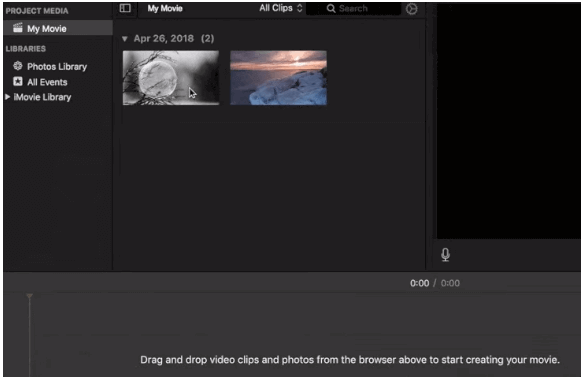A software window displayed in dark mode, likely an Apple application dedicated to movie or photo editing, occupies the screen. The interface features a black background with sections organized on the left side for easy navigation, including "My Movie," "Photos Library," "All Events," and "iMovie Library." Within the "My Movie" section, two videos are neatly presented and sorted by date, specified as October 26th, 2018. The first video showcases a stunningly professional cover shot of a vibrant blue glacier adjacent to a body of water, with the sun gorgeously setting in the background. The second cover shot offers an eerie, aesthetically captivating view of a seemingly enlarged moon, framed by stark, barren tree branches. This software, possibly iMovie, appears to support sophisticated movie editing capabilities, though the degree of its editing functionalities remains uncertain from the given description.